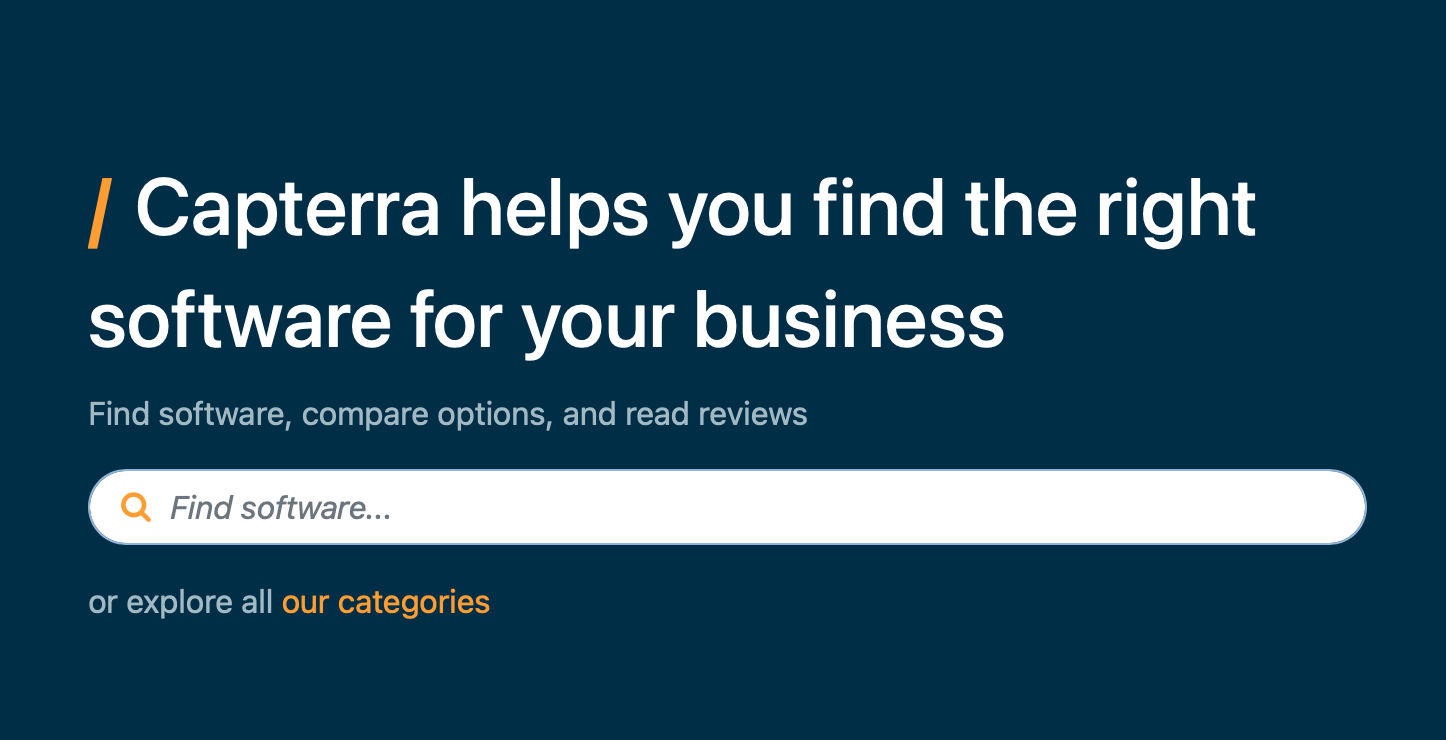The image displays a section of a website featuring a navy blue background. Dominating the center, there is a prominent phrase in white text that reads, "Capterra helps you find the right software for your business." Below this, a smaller tagline in grayish letters states, "Find software, compare options, and read reviews."

Beneath the tagline, an empty search bar invites user interaction with placeholder text that reads, "Find software..." To the left of the search bar, an orange magnifying glass icon indicates it is ready for user input. Just below the search bar, there is a call to action in white text: "Or explore all our categories," with "our categories" highlighted in orange.

The design includes an orange slash before the word "Capterra," adding a minimal yet distinctive visual element to the layout. The image is clean and focused on guiding users to either search for software directly or explore various software categories, emphasizing the website’s intent to assist in software discovery and comparison.